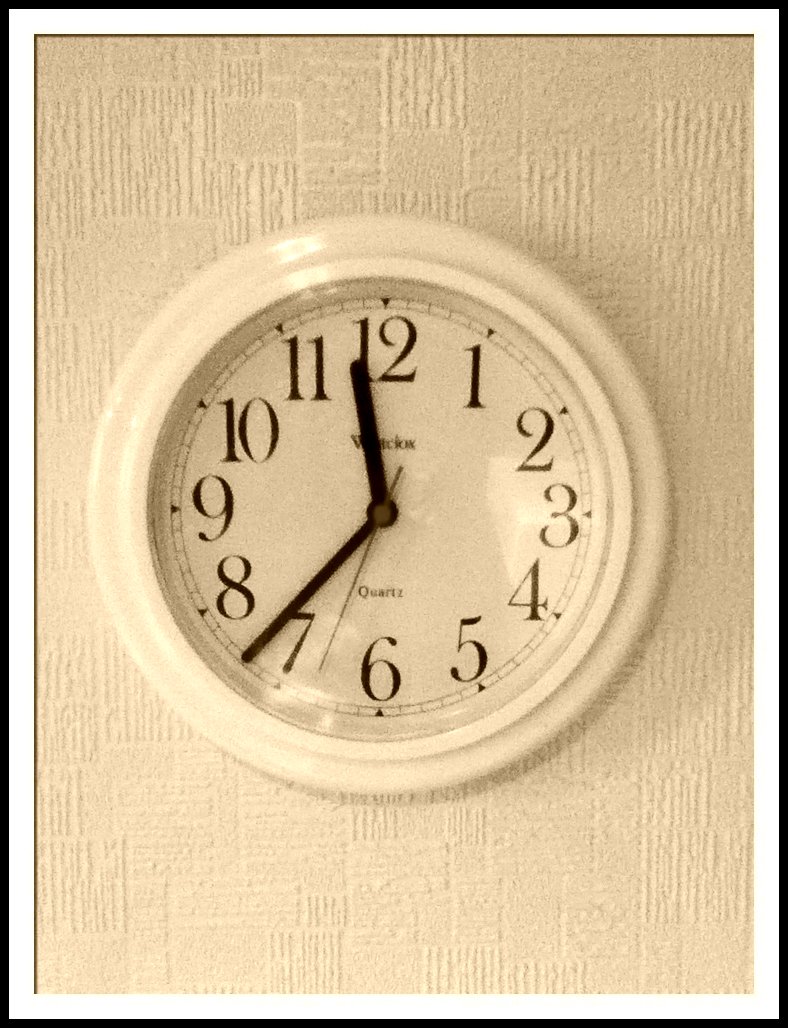The image features an illustration of a white, round wall clock mounted on a beige textured wallpaper, which is adorned with a pattern of vertical and horizontal lines. The clock has a thin black outer rim, followed by a whiter inner rim, and appears to be made of plastic. The face of the clock displays regular black numerals and black hands for the hours and minutes, while the second hand is slender and gold, with a gold circle at its base. The clock reads approximately 11:37, with the minute hand slightly past the 7. Below the number 12, there is some text, and just above the number 6, the word "quartz" can be seen. A slight shadow on the right side of the clock suggests a light source coming from the left, adding depth to the image.